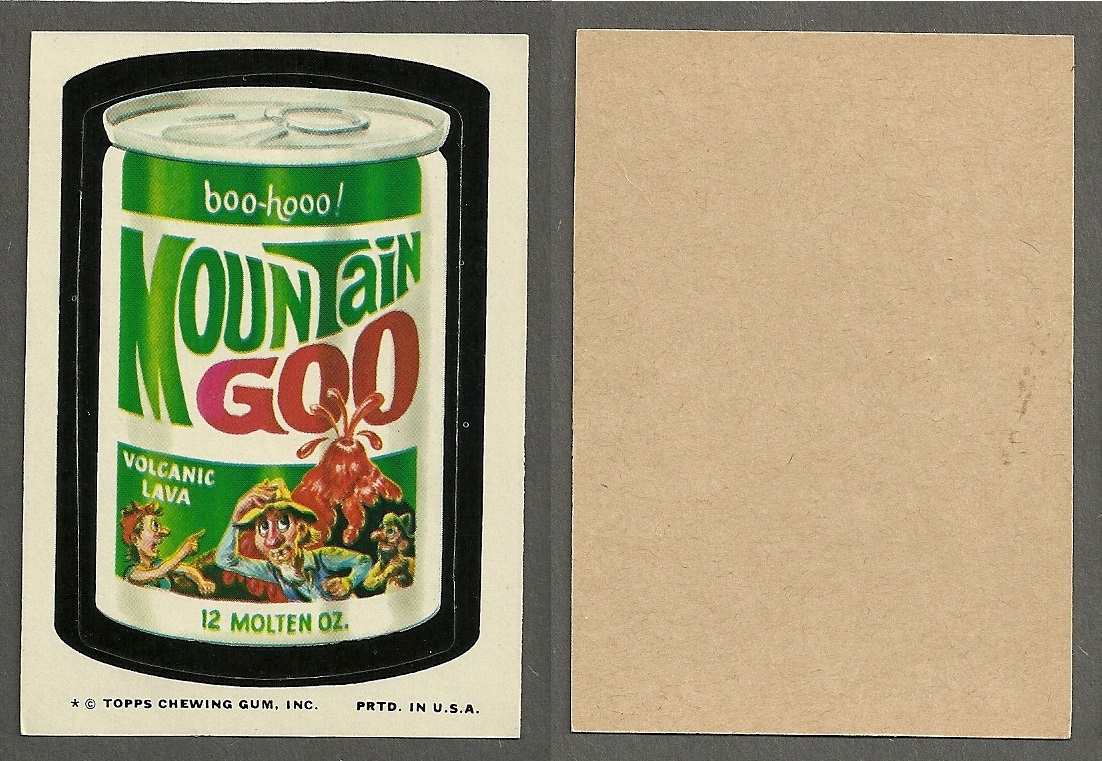The side-by-side images feature a front and back view of a collectible sticker. The first image showcases the front of the sticker, which has a vivid and playful illustration of a fictional soda can labeled "Mountain Goo," a humorous parody of the popular Mountain Dew drink. The can's label includes a green band with the text "Volcanic Lava," accompanied by a chaotic scene of people fleeing from an erupting volcano spewing red goo. The sticker's artwork is bordered in black, and the top of the can prominently features the phrase "Boo Hoo." The edges of the sticker are clearly defined, indicating where it can be peeled off. At the bottom, the words "Copyright Tops Chewing Gum Incorporated, Printed in the USA" are printed. The second image captures the sticker's back, which is entirely beige with a slight texture. Both photos are set against a medium gray background, providing a neutral contrast to the colorful details of the sticker.